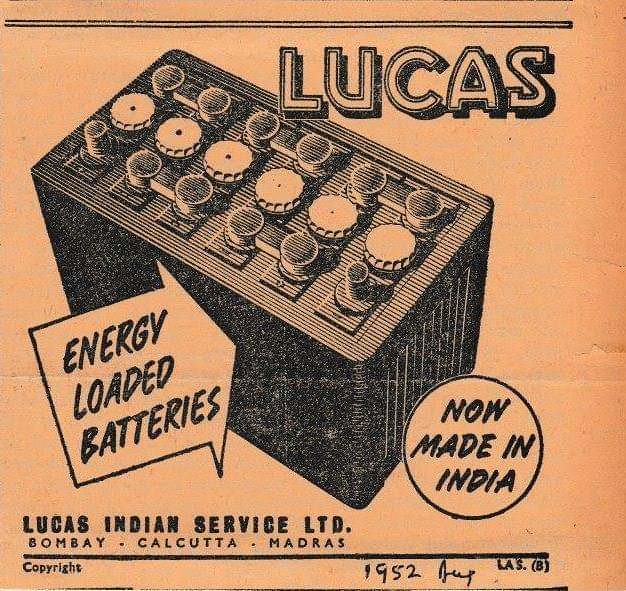This vintage 1952 advertisement, possibly from an old newspaper or magazine, features a light green, perhaps aged and yellowed, background. Central to the ad is an image of a car battery, depicted diagonally from the upper left to the lower right. Above the battery, bold black letters spell out "Lucas." An arrow pointing towards the battery reads "Energy Loaded Batteries." To the lower right of the battery, inside a circle, it declares "Now Made in India." Below this illustration, in large black print, the ad states "Lucas Indian Service Limited," followed by the cities "Bombay, Calcutta, Madras" in smaller print. An additional detail is noted at the bottom left: "Copyright August 1952" written by hand, adding to the nostalgic authenticity of the era.